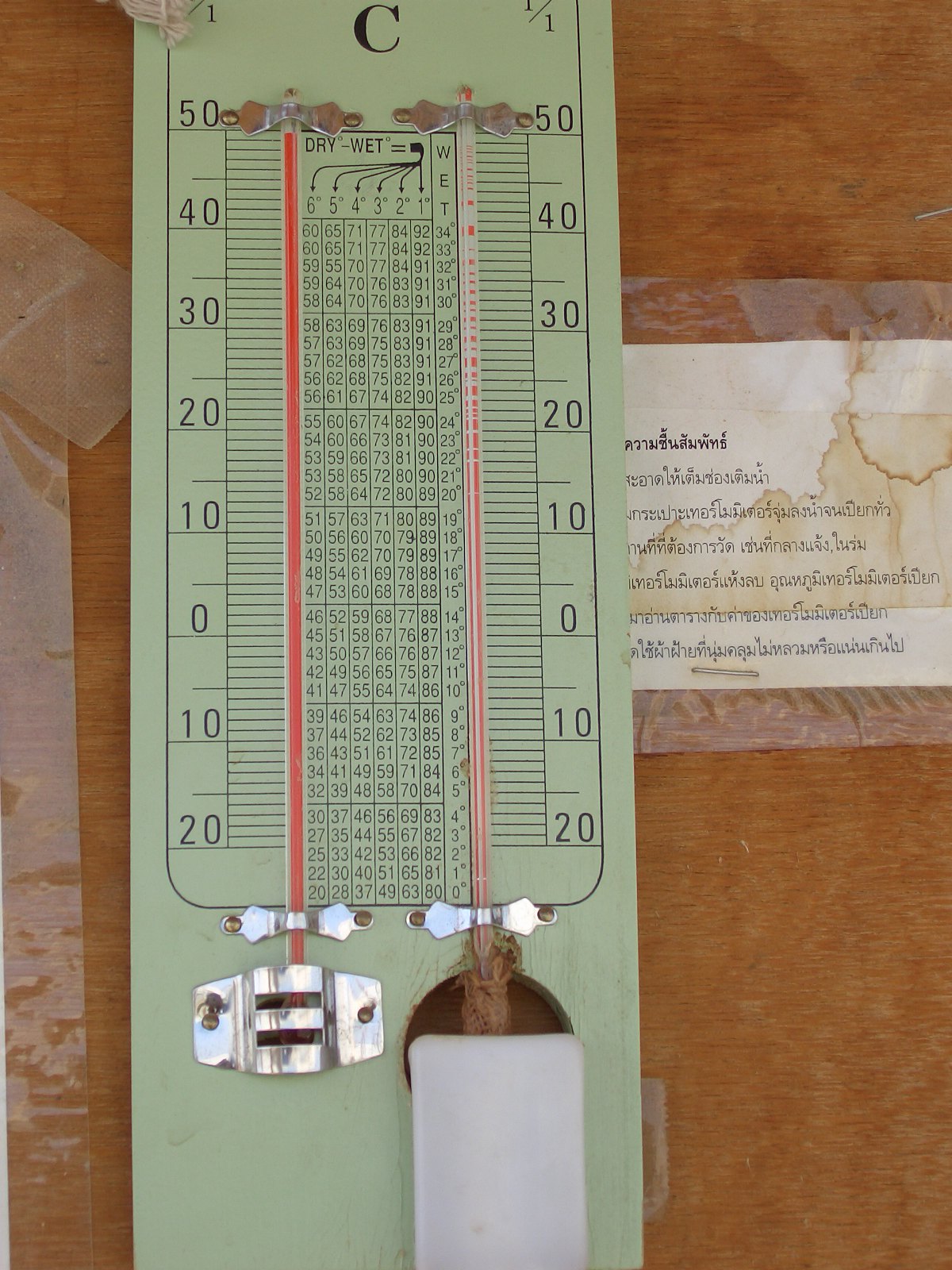This photograph features a detailed close-up of a traditional thermometer apparatus mounted on a green-colored board. The thermometer consists of two glass indicators filled with red liquid, securely held in place with silver clips that are affixed to the green backboard. The board prominently displays a temperature scale in black print, ranging from -20°C to 50°C, with numerals clearly marked at intervals (0, 10, 20, 30, 40, and 50). 

A large black letter 'C' is centrally positioned on the board, denoting Celsius. Between the two glass thermometers lies a table for additional temperature readings or notes. Adjacent to the green board is a piece of white paper, taped to a large timber notice board. This piece of paper contains lines of text in a Southeast Asian language, likely Thai, and bears visible brown stains, suggesting it has been in place for some time and is somewhat worn. The paper is attached using clear adhesive tape, further securing it to the wooden notice board.